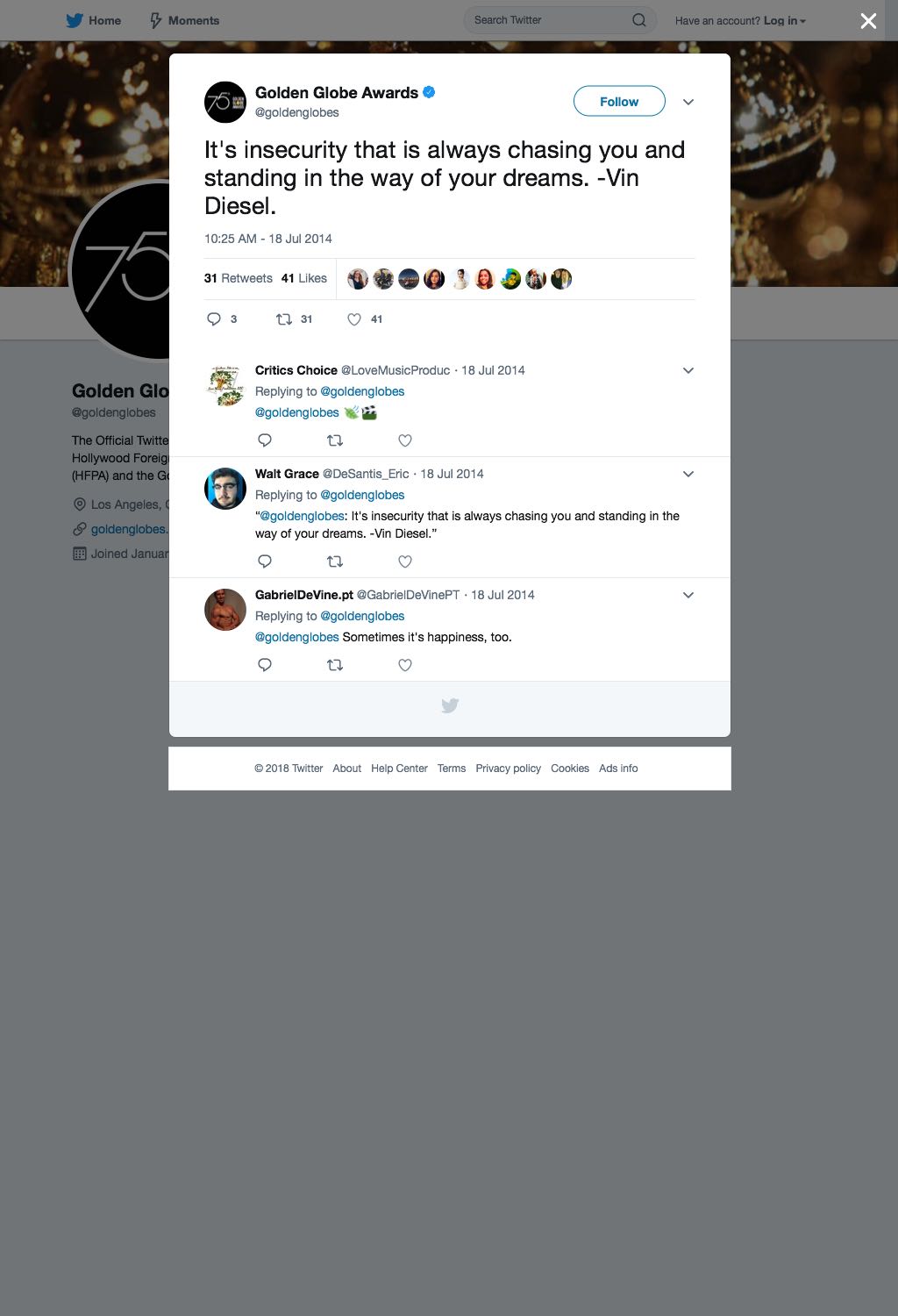This screenshot captures the Twitter homepage featuring a post. The background is predominantly gray, with the first page active. In the upper left corner, the iconic blue Twitter bird logo is visible. To the right of the logo are the navigation options: 'Home,' 'Moments,' and a search bar with the placeholder text 'Search Twitter.' Options for 'Have an account?' and 'Log in' are also displayed. 

In the upper right corner of the interface, a white ‘X’ symbol is present to close the page. A white overlay sits above the background. Within this overlay, in the upper left corner inside a circle, bold black text reads '75th Golden Globe Awards.' Directly beneath that text, the handle '@GoldenGlobes' is displayed alongside a small blue verified badge with a checkmark. 

In the upper right corner of the overlay, there is a 'Follow' button accompanied by a downward-facing arrow. The central content of the screenshot is a tweet that states: "It's insecurity that is always chasing you and standing in the way of your dreams. - Vin Diesel" posted at 10:25 AM on July 18, 2014.